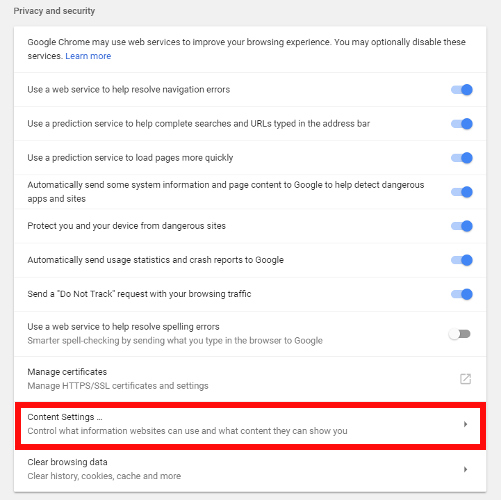This image is a screenshot of the "Privacy and Security" settings in Google Chrome, likely taken from a laptop screen. The interface is bordered by a light gray frame, which is thickest at the top and becomes progressively thinner on the sides and bottom. Inside this frame, the main content area is a white background adorned with black text.

In the top left corner, the gray border displays the label "Privacy and security" in black lettering. Directly beneath this, within the main white area, a heading states, "Google Chrome may use web services to improve your browsing experience. You may optionally disable these services," followed by a link in blue text that says "Learn more."

Below this heading is a list of toggleable options, allowing users to enable or disable various privacy and security features. There are a total of eight toggles, with the first seven switched on and the final one switched off. The last option reads, "Use a web service to help resolve spelling errors."

Additionally, the second-to-last option is emphasized with a red border around it and includes the description, "Content settings control what information websites can use and what content they can show you." Just above this, a non-toggleable option named "Manage certificates" appears, marked by a small square icon with an upward-right line extending from its corner.

At the bottom of the list, another non-toggleable option titled "Clear browsing data" is shown with an arrow pointing to the right, indicating further options or actions may follow upon selection.